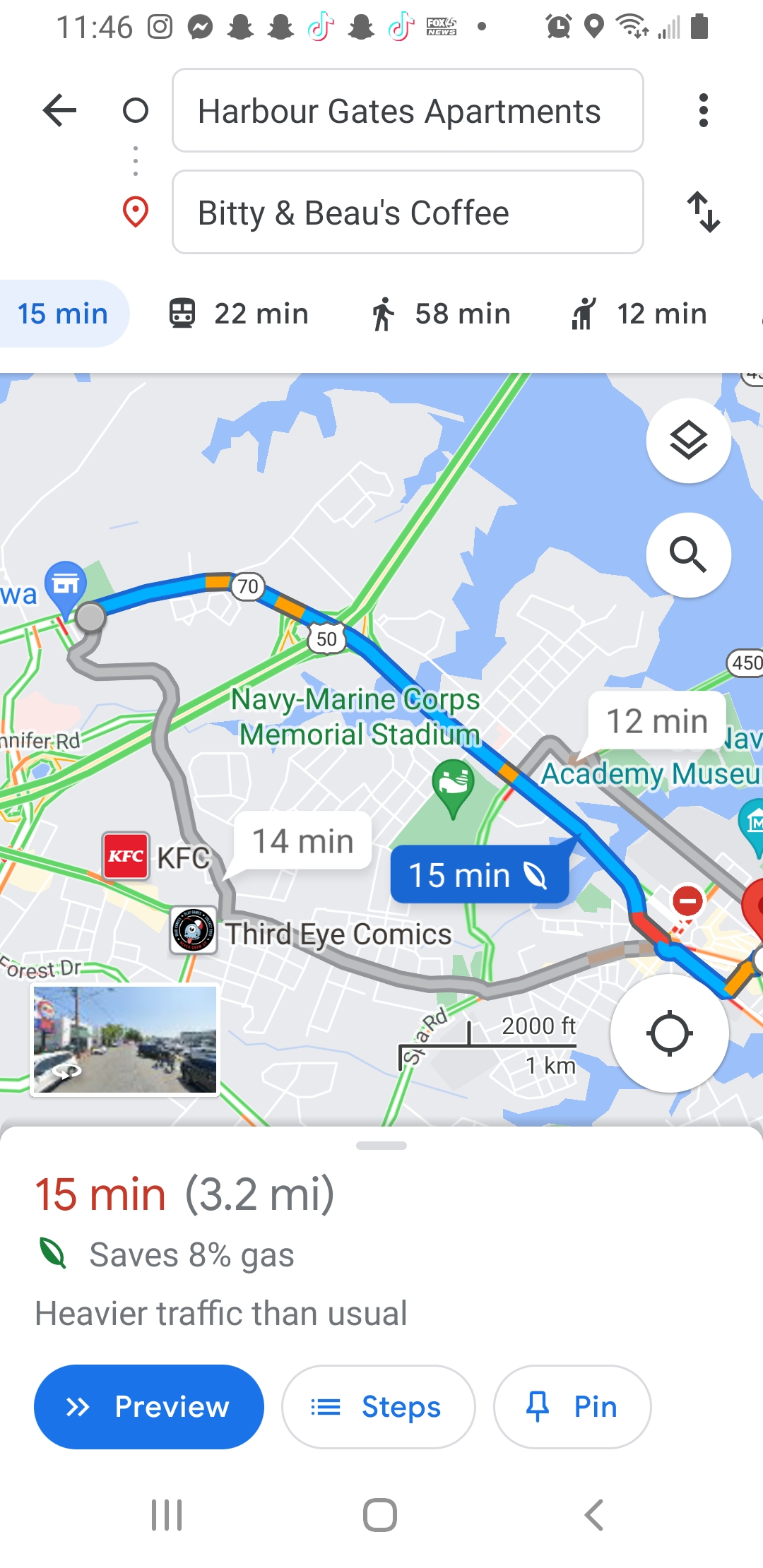This detailed screenshot from an Android smartphone displays Google Maps in use, navigating from Harbour Gates Apartments to Bitty and Beau's Coffee. The top of the screen indicates the current time as 11:46, with various notifications in the status bar, including Instagram, Facebook, Snapchat, and Twitter, along with system icons for an alarm clock, GPS location, Wi-Fi, signal strength (two bars), and a fully charged battery.

The central map screen shows a blue route line, interspersed with orange and red segments, indicating areas of heavier traffic leading to a 15-minute estimated travel time. This summary is shown in reddish-orange text alongside details that the route covers 3.2 miles. Additional route options are visible: driving (22 minutes), walking (58 minutes), and hailing a ride (12 minutes with a waving man icon). There's a small leaf icon next to the text suggesting an 8% gas saving for this route.

Icons and buttons at the bottom include options for a preview of the route, viewing steps, and pinning the route. The map itself is predominantly gray to represent the land, with blue waterways. Notifications also mention points of interest such as Third Eye Comics, Neonite, KFC, and the Navy-Marine Corps Memorial Stadium.